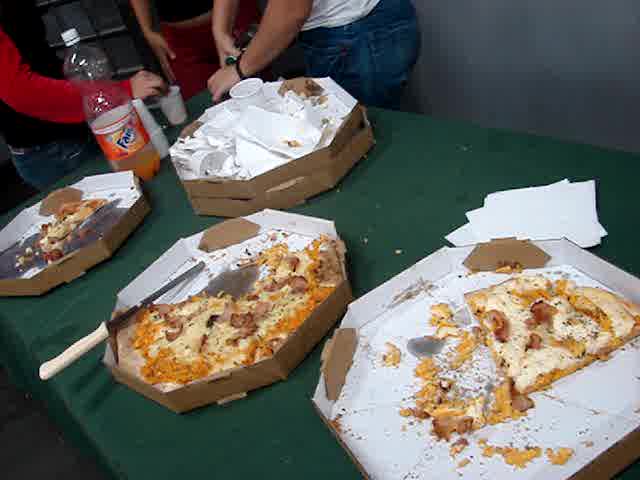This color photograph captures a scene with a green table adorned with a green tablecloth, situated against a gray wall. On the table, there are five pizza boxes in various stages of emptiness and disarray. 

One box, located at the lower right, has one and a half slices of pepperoni pizza left. Another box next to it is half-full with a medley of cheese, pepperoni, and sausage pizza. The third box appears to contain a single remaining slice. The fourth box seems mostly discarded, littered with crumpled up paper. Interestingly, there's a discrepancy regarding the total number of boxes—some descriptions mention four while others say five.

Also on the table, there’s a nearly empty bottle of orange Fanta soda accompanied by a stack of cups and a pile of white square napkins. A knife rests on one of the pizza trays.

In the background, partially visible, are the lower halves of three people standing behind the table. On the left is a man dressed in jeans and a white t-shirt, distinguished by a rope bracelet on his wrist. To his right stands a person whose hands suggest they might be a woman, wearing blue jeans with a long-sleeve red shirt and possibly a black vest. The third individual, identifiable by red pants, appears less discernible as they are cropped out by the image's edge.